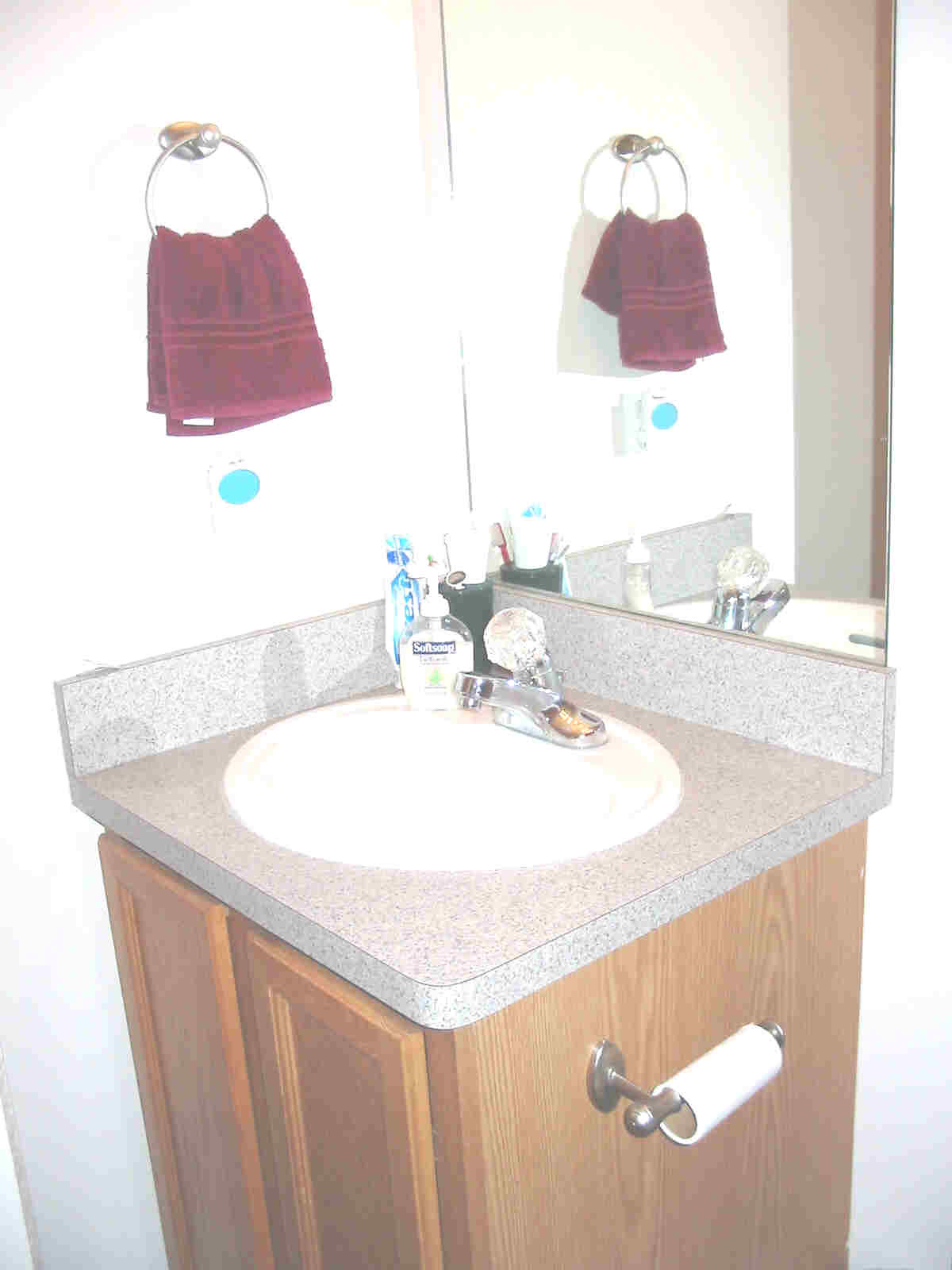In this cozy corner of a bathroom, a harmonious blend of functional and aesthetic elements creates a charming scene. A pristine white wall serves as the backdrop, adorned with a sleek, silver circular towel hanger. Draped over the hanger is a small red towel that features delicate stripes running halfway across it. Adjacent to the towel, a petite blue circle adds a splash of color to the wall.

A tall mirror stands nearby, reflecting not only the washcloth and the enigmatic blue circle but also enhancing the space’s sense of depth. Below the mirror, an elegant gray speckled countertop supports an oval-shaped white sink, its modern design complemented by a silver faucet. The faucet boasts a large white plastic handle for easy operation.

Adding to the practicality, a clear liquid soap dispenser with a white label and blue accent stands beside another small blue bottle, ready for use. The compact corner cabinet beneath the sink, crafted from light-colored wood, features two front doors that provide access to additional storage. On the side of this cabinet, a nearly depleted toilet tissue roll sits on a roller, emphasizing the well-used nature of this homely bathroom slice. The thoughtful arrangement of items in this bathroom corner combines functionality with subtle bursts of color and modern touches.